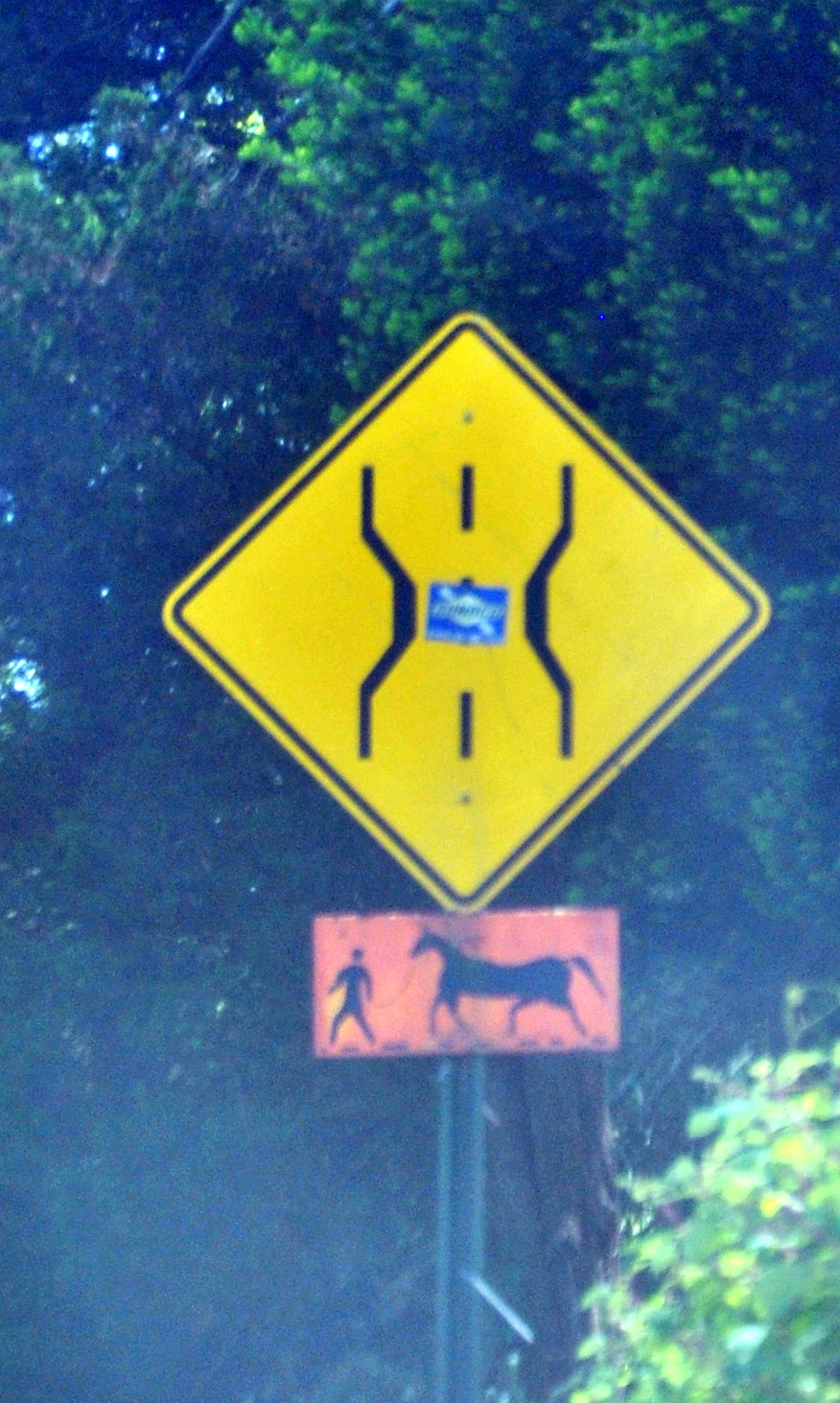In this bright and slightly bleached-out photograph, the focal point is a unique outdoor traffic sign set against a lush green backdrop of thick, dense trees and bushes. The main sign is a yellow diamond with a black border, featuring graphic lines that depict a roadway narrowing in the middle before widening again. Adding to the visual complexity, a blue rectangular Sunoco sticker is prominently displayed on the diamond sign. Below this is a smaller, rectangular sign with an orange-pinkish background, illustrating a person leading a horse on a leash. This sign appears to be hand-drawn or printed and suggests a shared path for pedestrians and horses. The entire assembly is mounted on a metal pole, standing out vividly against the verdant background.